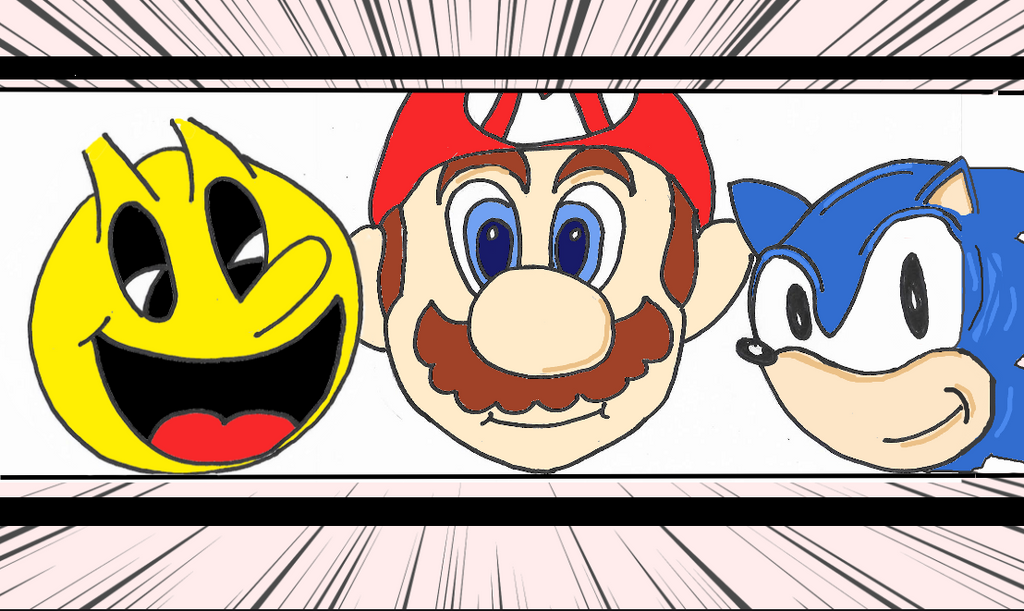This image showcases a marker drawing of three notable video game characters grouped together on a white background. On the left is Pac-Man, depicted with a yellow circular head, wide-open mouth, and red tongue, slightly deviating from the traditional look with added features like expressive eyes with whites. In the center is Mario from the Mario Brothers game, characterized by his big blue eyes, red mustache, sideburns, eyebrows, and his iconic bright red cap emblazoned with a red 'M'. To the right is Sonic the Hedgehog, presented in his classic blue color with big black eyes and a small black nose. The simplicity of the white background is interrupted by black and pink striped designs at the top and bottom, adding a decorative touch to the drawing. The characters appear somewhat crudely rendered, reminiscent of artwork by a younger artist or someone new to the industry.